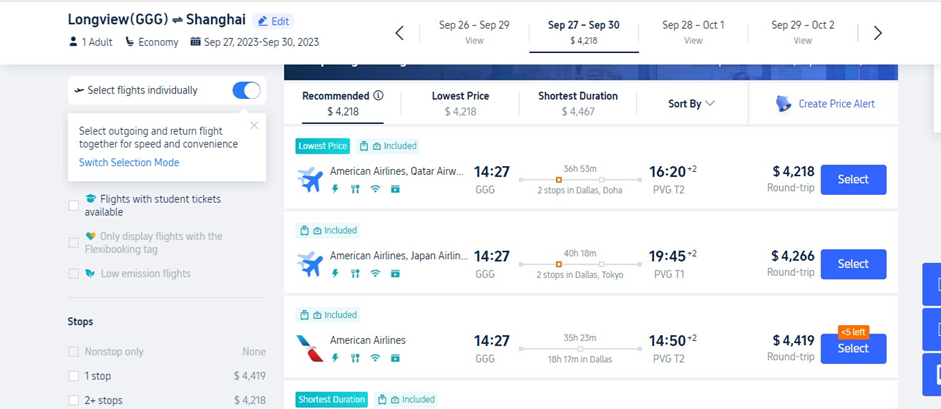The image displays a flight booking interface with several options and details visible. At the top, bold text reads "Longview, GGG, Shanghai, one adult economy, September 27th, 2023 through September 30th, 2023." Below this, interface options include "Select flights individually," and "Select outgoing and return flight together for speed and convenience," with an option to "Switch selection mode." There is also a section titled "Flights with student tickets available," followed by options to display only flights with the FlexiBook tag and low-emission flights.

On the right side, search results appear, prefaced with categories like "Recommended $4,218," "Lowest price $4,218," and "Shortest duration $4,467." Additionally, there is a "Sort by" tab and a button to "Create a price alert." Notable entries include a highlighted lowest price option: "American Airlines, Qatar Airways, $1,427, GGG to PVG, T2," indicating the flight costs and details for travel between Longview (GGG) and Shanghai (PVG T2).